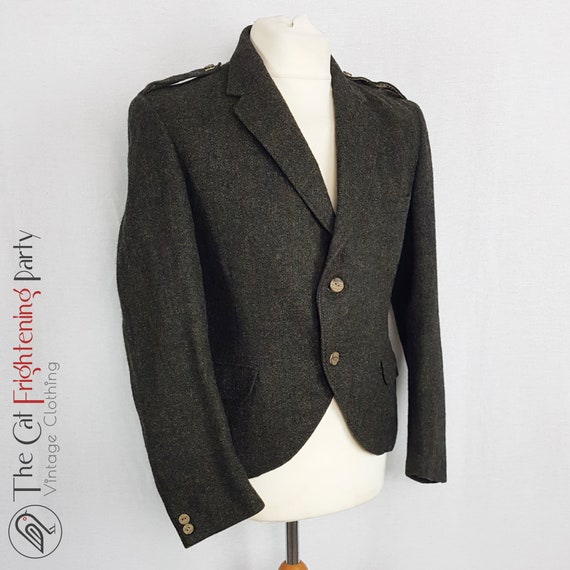The photograph features a men's dark gray jacket displayed on the upper torso of a white mannequin, against a gray background. The jacket, which combines elements of a hunt coat and a dressage coat, is distinctly styled to hit at the hips and includes two ivory bone buttons fastened at the front. It also features military-inspired shoulder lapels and two false pocket flaps. The sleeves are accented with two bone buttons each. Running vertically along the left edge of the image, there's a title that reads "The Cat Frightening Party Vintage Clothing," accompanied by a logo featuring a contemporary bird, likely an owl or robin, with one orange eye. The steel rod supporting the mannequin is also visible, emphasizing the minimal and focused display. The overall aesthetic suggests the image could be part of a catalog advertisement or a promotional brochure for vintage clothing.